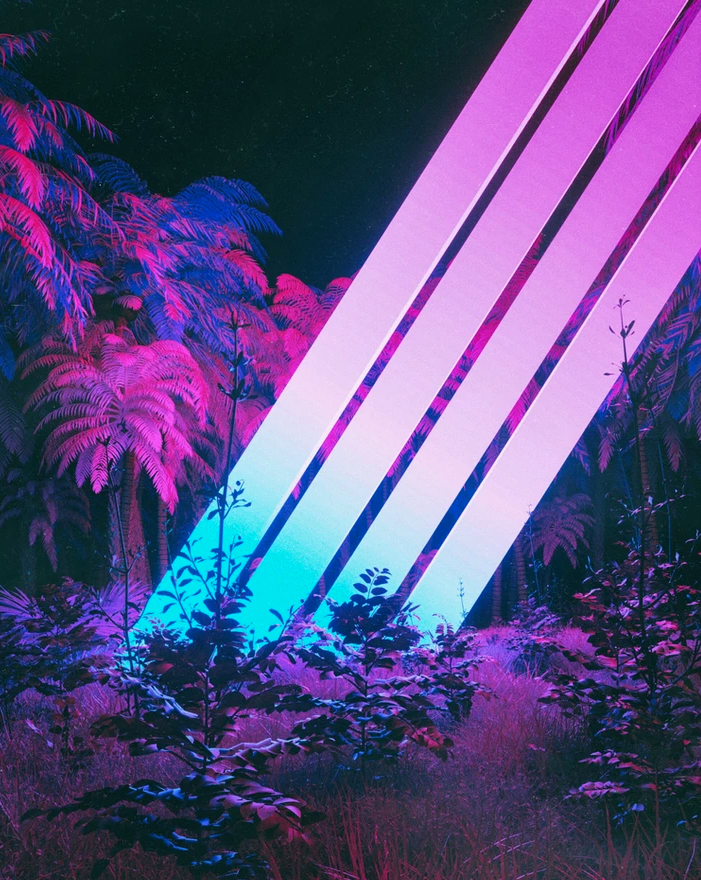In this vivid, two-dimensional landscape image, a series of purple, pink, and neon blue hues dominate the scene, creating a visually striking 80s-inspired aesthetic. The foreground features several bushes and patches of thin grass illuminated by a purple light. Encircling the scene, palm trees form a perimeter against a pitch-black sky, which, on clear nights, may reveal faint stars. Central to the image are four evenly spaced diagonal bars, starting from the upper right and stretching toward the lower left. These bars, approximately 10% of the image's width, transition in color from purple at the top through bright white in the middle, and culminating in a vivid blue at their base where they meet the ground. The overall effect is a dramatic spectacle of neon-inspired artistry, with the diagonal stripes adding a dynamic intersecting element to the lush, shadowy foliage.